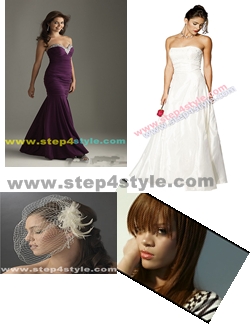The image is composed of a collage featuring four distinct photographs, each showcasing different women in various fashion-focused poses and attire. 

In the top left corner, a woman with long black hair is wearing a deep purple mermaid-style strapless gown, adorned with a sequined or silver sweetheart neckline that forms a V-shape down to her knees, flaring at the bottom. This elegant dress highlights her bare chest and arms. 

To the right, there's an image of a woman in a sleek, white strapless dress, evocative of a wedding dress. Her hair is styled up in a bun with a few wisps loose, and she holds a rose or similar object. The dress, made from a satiny material, fits snugly around her chest and flares out towards the bottom. She casts her gaze downward, adding a dramatic flair to the composition.

In the bottom left corner, the focus is on a woman's upper neck and face adorned with a delicate veil featuring a sprig of feathers on the side. Her hair is partially covered by this bridal-like netting, reminiscent of a fascinator without the visible hat.

Finally, the bottom right picture shows a woman with reddish-brown hair, long bangs partially covering her eyes, and peachy lipstick. She rests her right arm on her cheek and wears a black and white striped shirt, reminiscent of a style icon like Rihanna. Her image is slightly skewed compared to the others.

Each photograph includes the website "www.step4style.com" in various colors and placements, unifying the collage toward a fashion theme.